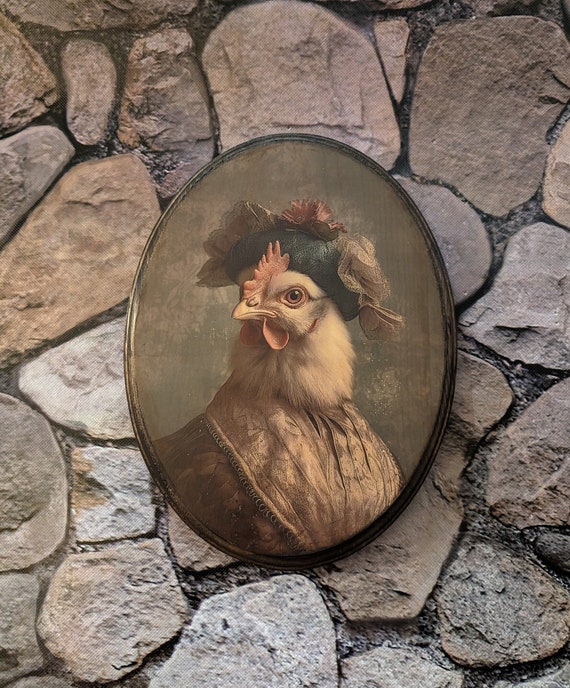The image is a detailed portrait of a hen presented in an oval-shaped locket. The hen wears an ornamental light green hat adorned with fabric curls and small flowers. Its attire is a goldish, puffed robe or dress, accented with dark fabric running down, and features a collared vest with lacy white decorations. The hen's side profile shows it looking into the viewfinder with one eye. The background of the locket image is dark gray with hints of blue. The locket itself has a light black border and appears worn and rusted. This locket is set against a backdrop of variously colored stones, ranging from light beige to dark gray, intricately connected with no gaps in between.